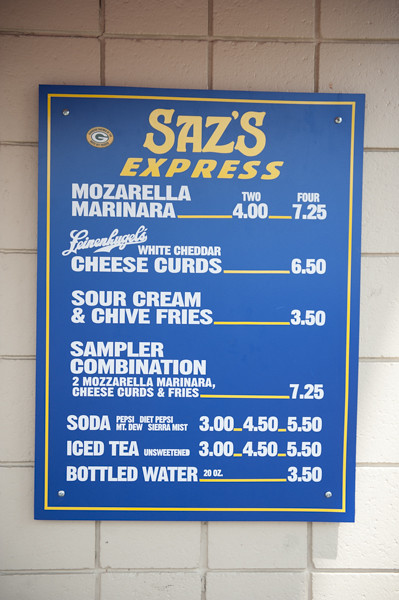The image features a detailed menu sign mounted on a tile wall that transitions from a brownish-pink hue at the top to a darker shade of white on the left side and a pure white on the right. The menu is displayed on a blue, rectangular sign with an inner orange and yellow outline. The sign appears to be affixed to the wall with two rivets.

In the top left corner of the sign, there's a yellow circle with a white "G" in the center and some small, unreadable text surrounding it. Below this circle, the menu reads "Saz Express" in yellow, followed by "Mozzarella Marinara" in white.

Subsequently, the menu lists:
- Mozzarella Marinara: $2.00 for one serving, $4.00 for two servings, and $7.25 for a combination with another item that is unreadable.
- White Cheddar Cheese Curds: $6.50
- Sour Cream and Chive Fries: $3.50
- Sampler Combination: Includes Mozzarella Marinara, Cheese Curds, and Fries for $7.25.

The beverage section lists:
- Soda options (Pepsi, Diet Pepsi, Mountain Dew, Sierra Mist): $3.00 for regular, $4.50 and $5.50 for larger sizes.
- Iced Tea (unsweetened): $3.00 for regular, $4.50 and $5.50 for larger sizes.
- Bottled Water (20 ounces): $3.50

Each item and price on the menu is neatly separated by a yellow line.